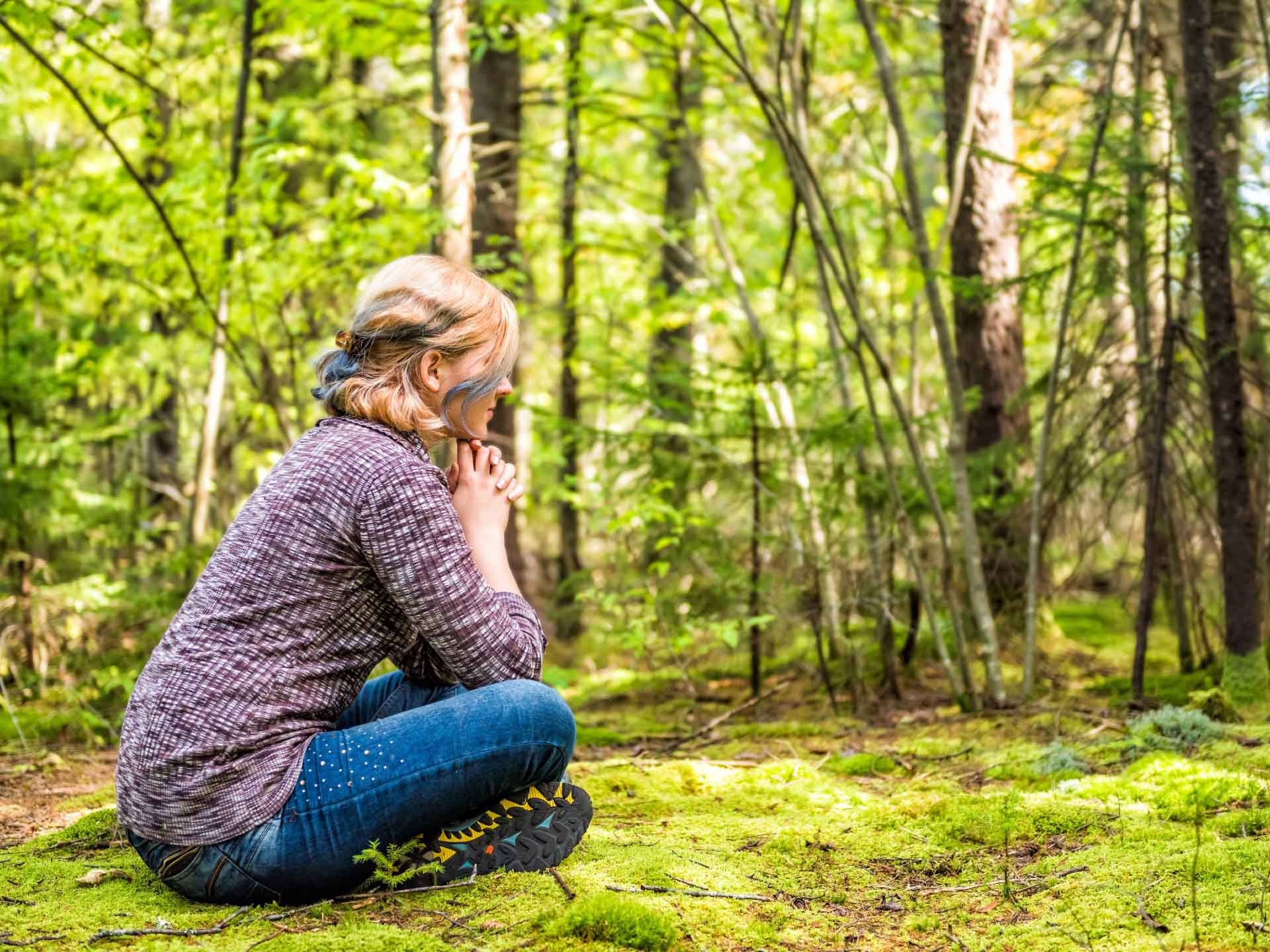In the image, a young woman is sitting in a serene, vibrant forest, positioned on the left side of the frame. She's seated cross-legged on a bed of lush moss, surrounded by tall trees with sunlight filtering through their canopy. Her attire includes blue jeans with decorative diamonds near the pockets, hiking shoes with distinct yellow spikes on their soles, and a textured, purplish-gray sweater-like shirt. The woman has blonde hair streaked with blue highlights, which is clipped back from her face. She is gazing off to the right with her elbows resting on her knees, hands clasped in a manner that resembles a prayer stance. The forest backdrop, rich with greenery and natural light, adds to the tranquil and vibrant atmosphere of the scene.